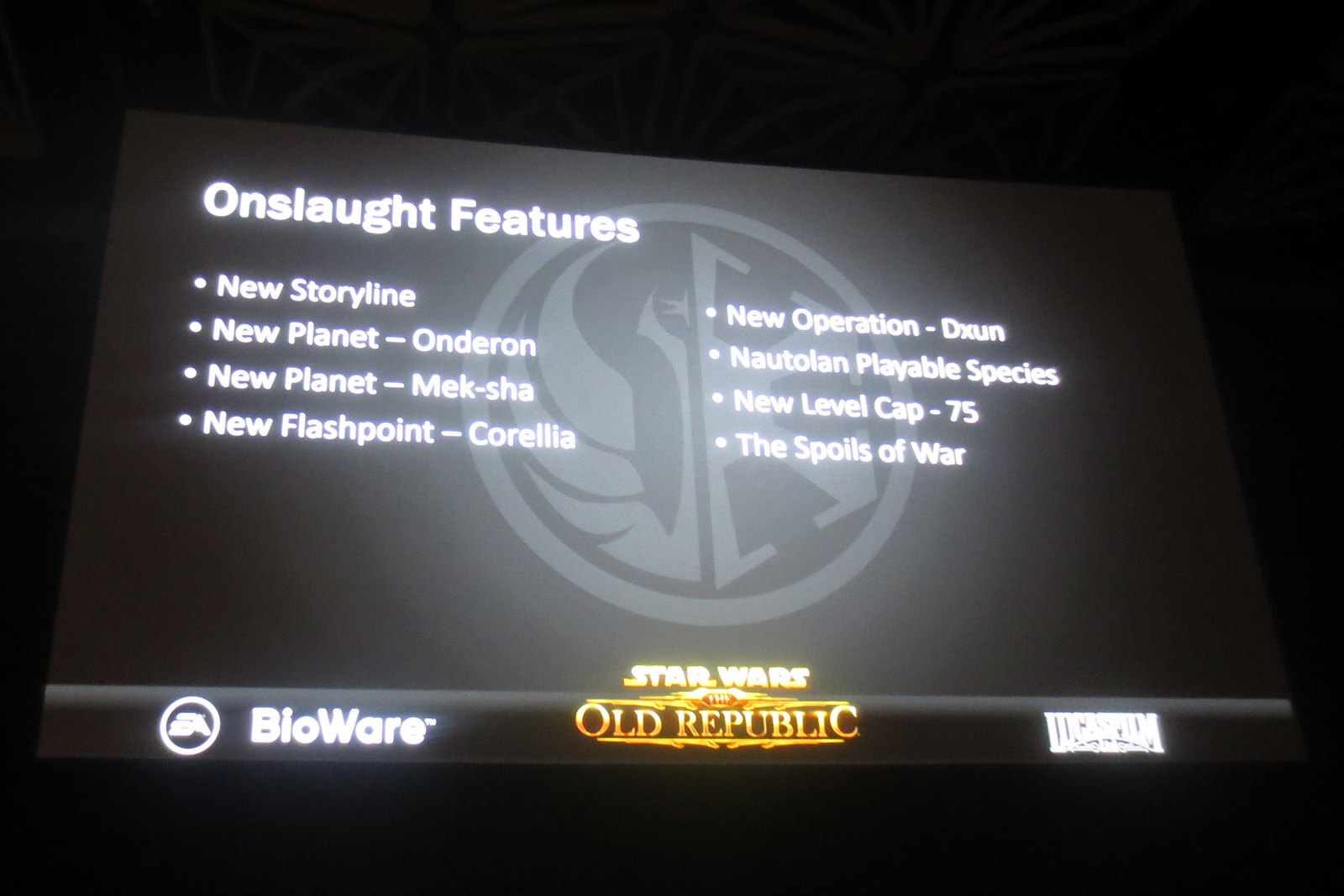This image appears to be a screenshot taken from a computer screen, depicting information about a Star Wars-themed video game called Star Wars: The Old Republic, developed by BioWare in partnership with Lucasfilm. The entire background is black, with a dark gray rectangular area in the center, making it look like a close-up of a computer monitor or a projection on a screen. At the top of the screen, in large white letters, it says "Onslaught Features." The text lists several new features in white, including "New Storyline," "New Planet: Onderon," "New Planet: Meksha," "New Flashpoint: Corellia," "New Operation: Dxun," "New Playable Species," "New Level Cap: 75," and "The Spoils of War." At the bottom left, the BioWare logo is visible alongside the EA symbol. In the middle of the image, the title "Star Wars: The Old Republic" is displayed prominently in gold letters, and to the right of this title, the Lucasfilm logo is also visible. This image likely serves as a promotional screenshot outlining updates and new features for the video game.